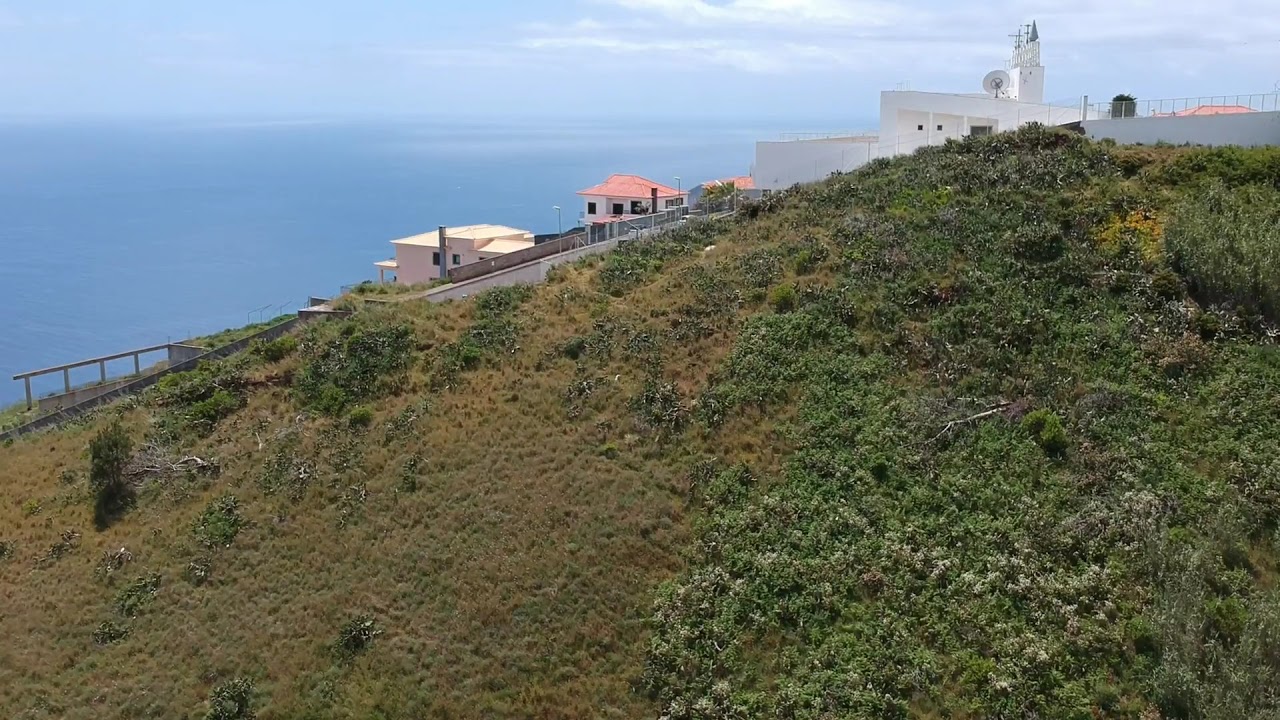The image depicts a high vantage point, likely captured by a drone, showcasing a scenic landscape. In the foreground, there's a sprawling, bush-covered hill with a mix of yellow and brown vegetation, indicating a dry season, perhaps summer or early autumn. The hill is dotted with various trees and plants, transitioning from lush greenery on the right to more yellowish hues on the left. Atop and along this hill are several buildings, with a prominent large white building on the right and another white house with an orange-pink roof in the middle. Nearer to the ocean on the left side, there's an off-yellow, almost white, house. One notable building features an antenna on its roof, suggesting modern amenities. In the background, a vast expanse of blue ocean stretches out, merging with an overcast, slightly cloudy sky, giving the image a serene yet hazy ambiance. The landscape, with its Mediterranean architectural style, hints at a possible location in Spain, Italy, or Greece.